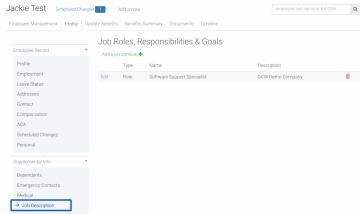The image depicts a small screenshot of a website with a white background. In the top left corner, the text "Jackie Test" is displayed in black letters. To the right of this text, there are some blue letters that are difficult to discern due to the image's size. Adjacent to these letters, on the right-hand side, is a search bar.

Below this header section, there are multiple tabs for navigation, although the text on these tabs is not legible in the image. On the left side of the page, there’s an additional vertical menu with a light blue background and various clickable tabs. At the bottom of this menu, one item is outlined in a darker blue.

On the main area of the page, to the right of the vertical menu, the heading "Job Roles, Responsibilities, and Goals" is prominently displayed at the top. Following this heading, there are some green words, with further sections labeled "Type," "Name," and another unreadable heading. Below these sections, there is at least one listed item, although the specifics are again difficult to discern. To the far right of the listed item, there’s a red trash can icon, suggesting an option to delete the item. The overall layout appears to be a functional interface where users can view and manage their job-related roles and responsibilities.